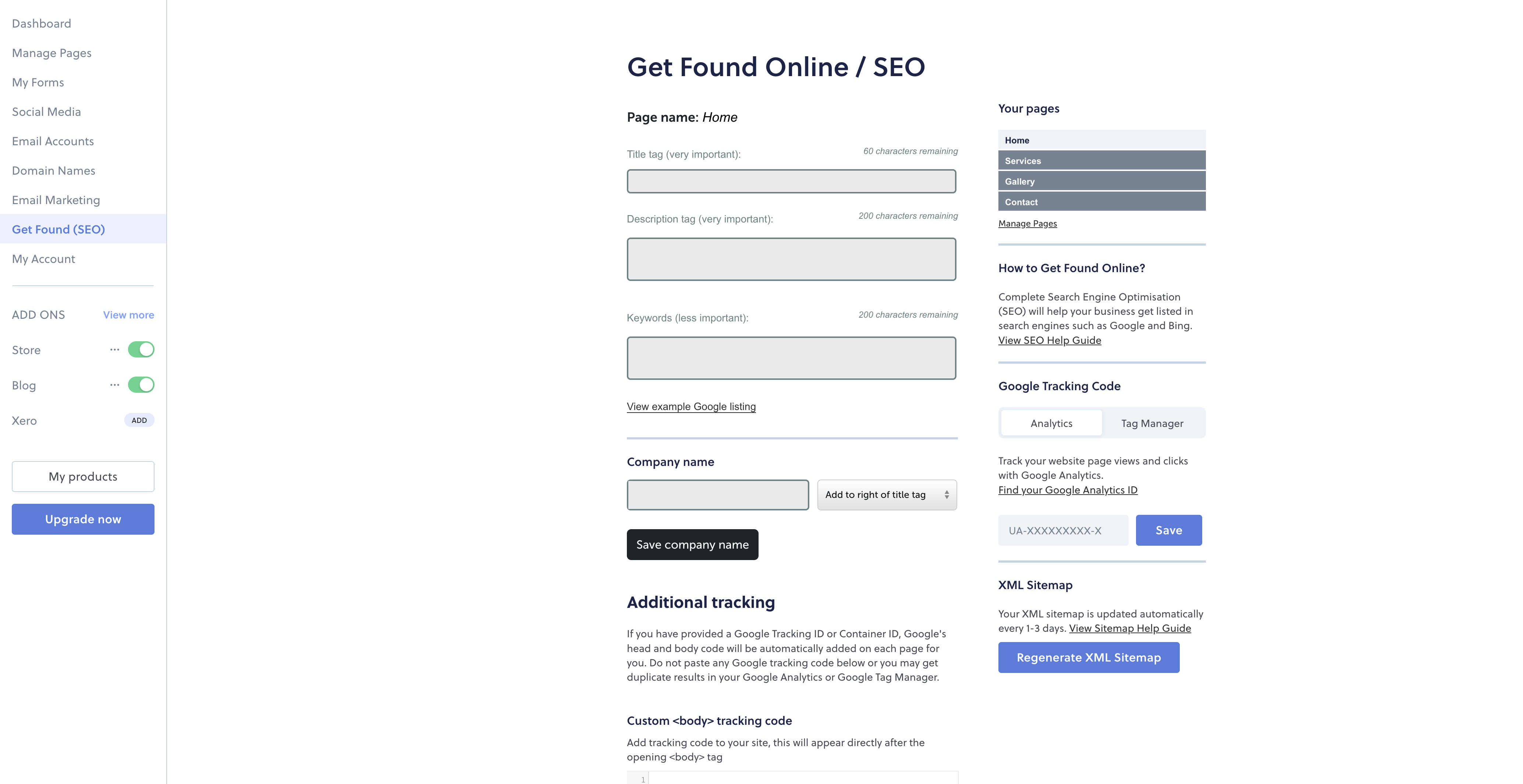This image captures a detailed view of a website interface, possibly a dashboard. On the left side, there's a vertical menu panel with a white background and predominantly gray text. The menu items listed include: Dashboard, Manage Pages, My Forms, Social Media, Email Accounts, Domain Names, Email Marketing, Get Found, and SEO. This section also features some highlighted text in blue, such as "My Account," "Add-ons," and a "View More" button.

Further down, there are two green oval icons with white circles and dots inside, labeled "Score" and "Blog". Additionally, there are sections noting "Zano" and "Add". Below this, there's "My Products" in black and white, and a prominent "Upgrade Now" button in blue and white.

Switching focus to the right side of the image, a heading in navy font reads "Get Found Online / SEO". This area is designated as "Page Name: Home" and includes three gray text boxes with adjacent gray font descriptive labels. Below these, there’s a section titled "View as Sample Google Listing".

Further down, there is an input field labeled "Company Name" with a gray box containing black text. Beneath this, a black box with white text offers an option to "Save Company Name". 

Continuing down, there's a section with a navy font heading titled "Additional Tracking". This area provides instructions for entering a tracking ID number. Below this is a section titled "Custom Tracking Code" with a short explanatory text.

Further right, a section titled "Your Pages" features four gray sub-menus. Below this, "How to Get Found Online" is presented with a paragraph of gray text. Next, there’s a heading "Google Tracking Code, Analytics, Manager" followed by a directive to "Track your website page views and clicks with Google Analytics" and a prompt to "Find your Google Analytics ID". There's also a blue and white "Save" button.

Finally, at the bottom, the text "XML Sitemap" appears alongside a brief gray sentence, with a blue and white "Regenerate XML Sitemap" button below it.